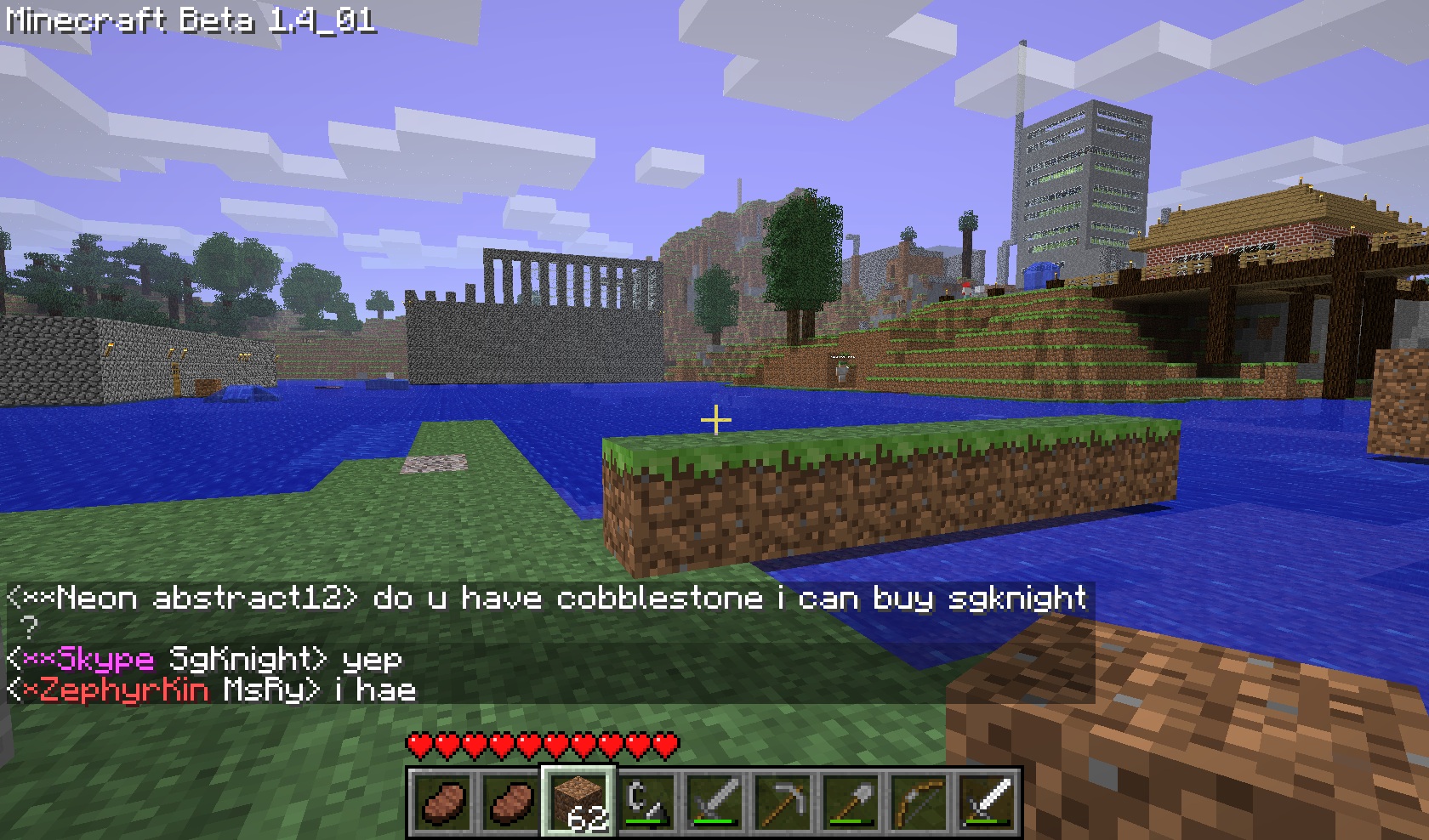The image is a detailed screenshot from the video game Minecraft, identified by the text "Minecraft Beta 1.4_01" in the upper left corner. The sky is a light purple shade with pixelated gray clouds, contributing to the classic Minecraft aesthetic. Below the sky, there's a tree line composed of various green, pixelated trees. In the middle ground, a cityscape features pixelated buildings, including a tall, gray structure with yellow lighting, and a brick wall that extends down a hill towards a body of water. On the right side, a set of brick steps leads from the water to the large gray building. In the foreground, there is green pixelated grass and a small bridge constructed of dirt blocks with green tops extending into the water. The bottom of the image shows a chat log where one user, NeonExtract12, asks, "Do you have Cobblestone? I can buy SG Knight?" followed by a response from SkypeSGKnight, "Yep." Another user named ZephyrKinMSRY adds, "I-H-A-E." Below the chat is a rectangular inventory bar displaying various items, including pieces of meat, wooden blocks, and several Minecraft tools. The scene comes together to encapsulate a vibrant and bustling area within the blocky universe of Minecraft.